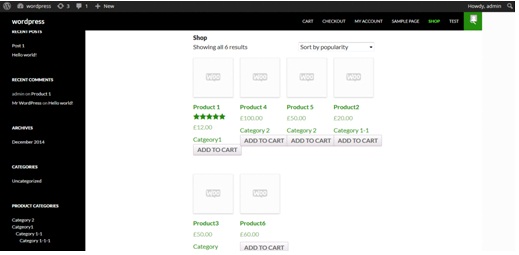A detailed caption for the image provided could be as follows:

"A landscape-oriented, color screenshot of a user's computer screen showcasing their web browser open to a WordPress online store page. The site appears somewhat blurry and pixelated, making it difficult to discern finer details like command buttons or the system clock. At the top of the browser, visible tabs include 'Cart,' 'Checkout,' 'My Account,' 'Sample,' and 'Shop.' The user has accessed the 'Shop' tab and the display shows a search result page with options to sort products by popularity or other filters. The interface indicates 'Showing all 6 results,' with product listings visible below. Specific listings include Product One, rated five out of five stars and priced at £12, and Product Four priced at £100, among others such as Product Two at £20 and Product Five at £50. Each product listing features an 'Add to Cart' button for purchase actions."